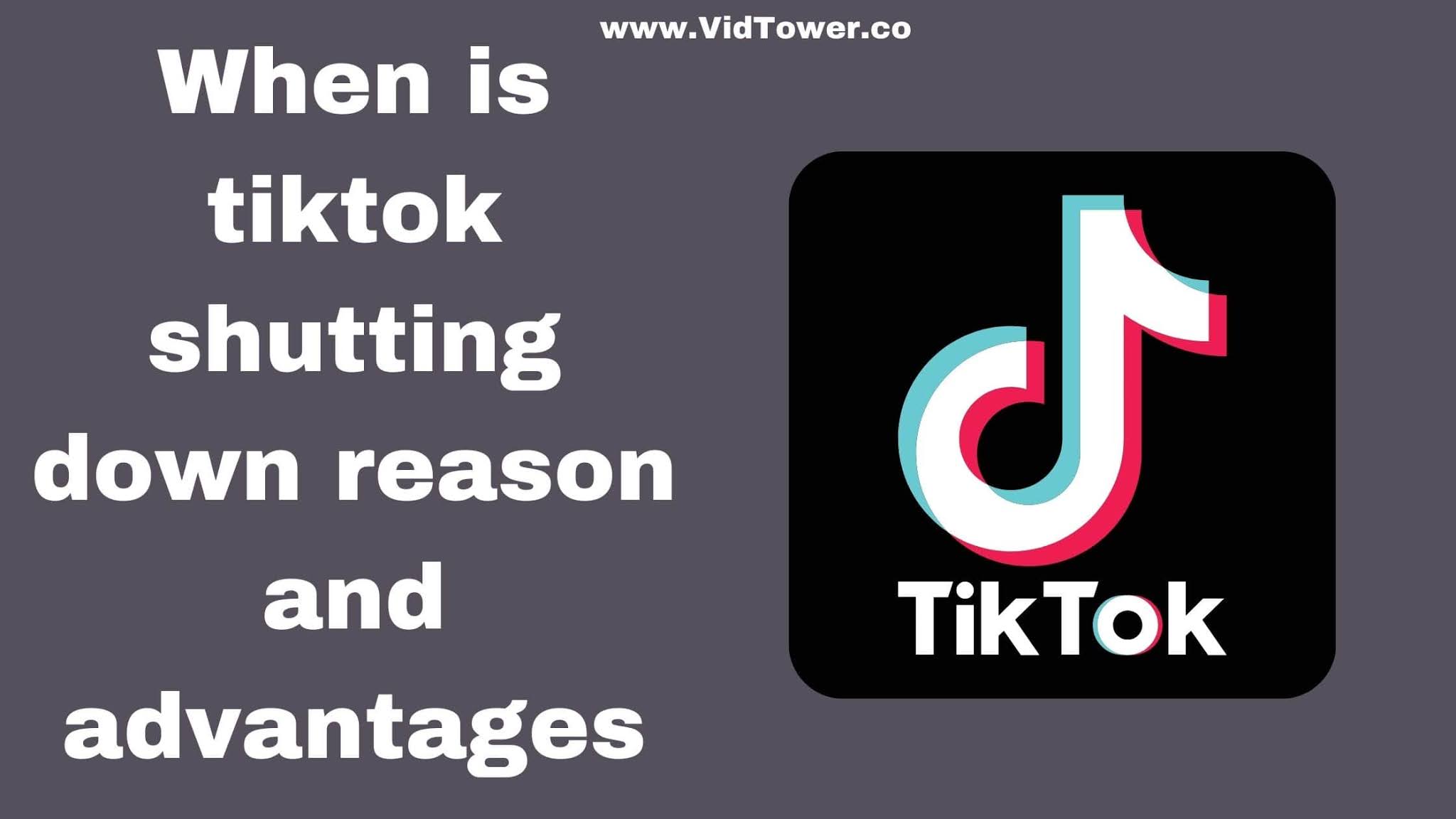This image features a sign related to TikTok. The background is predominantly gray, creating a neutral canvas for the text and graphics. At the top of the sign, in very small white print, is the URL: www.vidtower.co. 

Prominently displayed on the left side in larger white print is the question (sans question mark): "When is TikTok shutting down? Reason and advantages?"

Centrally positioned is a large representation of the TikTok app icon. The icon has a black, square background with rounded edges, giving it an authentic app-like appearance. At its center is the familiar TikTok logo, which consists of a stylized musical note in a blend of teal, white, and reddish hues. Below the musical note, the text "TikTok" is displayed, with a distinctive typography: 'Tik' is written with a capital 'T' followed by lowercase 'i' and 'k,' and 'Tok' begins with a capital 'T' followed by lowercase 'o' and 'k.'